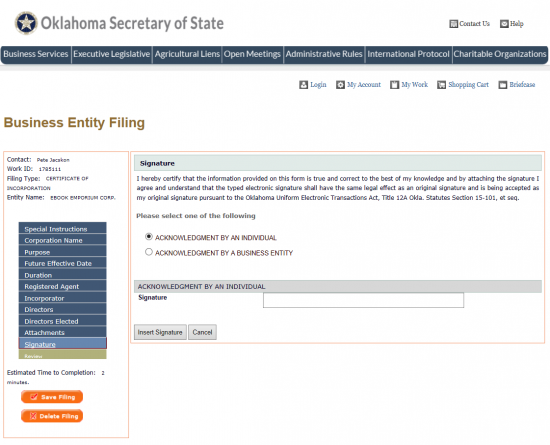The image depicts a webpage from the Oklahoma Secretary of State's website. In the upper left corner, the logo features a star encircled by a mottled pattern of light brown and white, set against a blue background with an outline. On the right side of the header, text reads "Contact Us" and "Help." A horizontal blue navigation bar with white text extends from the left, listing sections such as Business Services, Executive Legislation, Agricultural Liens, Open Meetings, Administrative Rules, International Protocol, and Charitable Organizations. 

To the right of the navigation bar are options for account management, including "Log In," "My Account," "My Work," "Shopping Cart," and "Briefcase." Below the navigation bar, on the left, a section titled "Business Entity Filing" appears in a light tan color. This section displays details for "Contact Pete Jackson" with a Work ID of "1795111" and type "Filing." Specifically, it pertains to a "Certificate of Incorporation" for the "eBooks Emporium Corporation."

The navigation area beneath this section includes links such as Special Instructions, Corporate Name, Purpose, Future Effective Date, Duration, Registered Agent, Incorporator, Directors, Directors Elected, Attendance, and Signature. At the bottom, two orange buttons labeled "Estimated Time to Completion: One Minute," "Save Filing," and "Delete Filing" are prominently displayed.